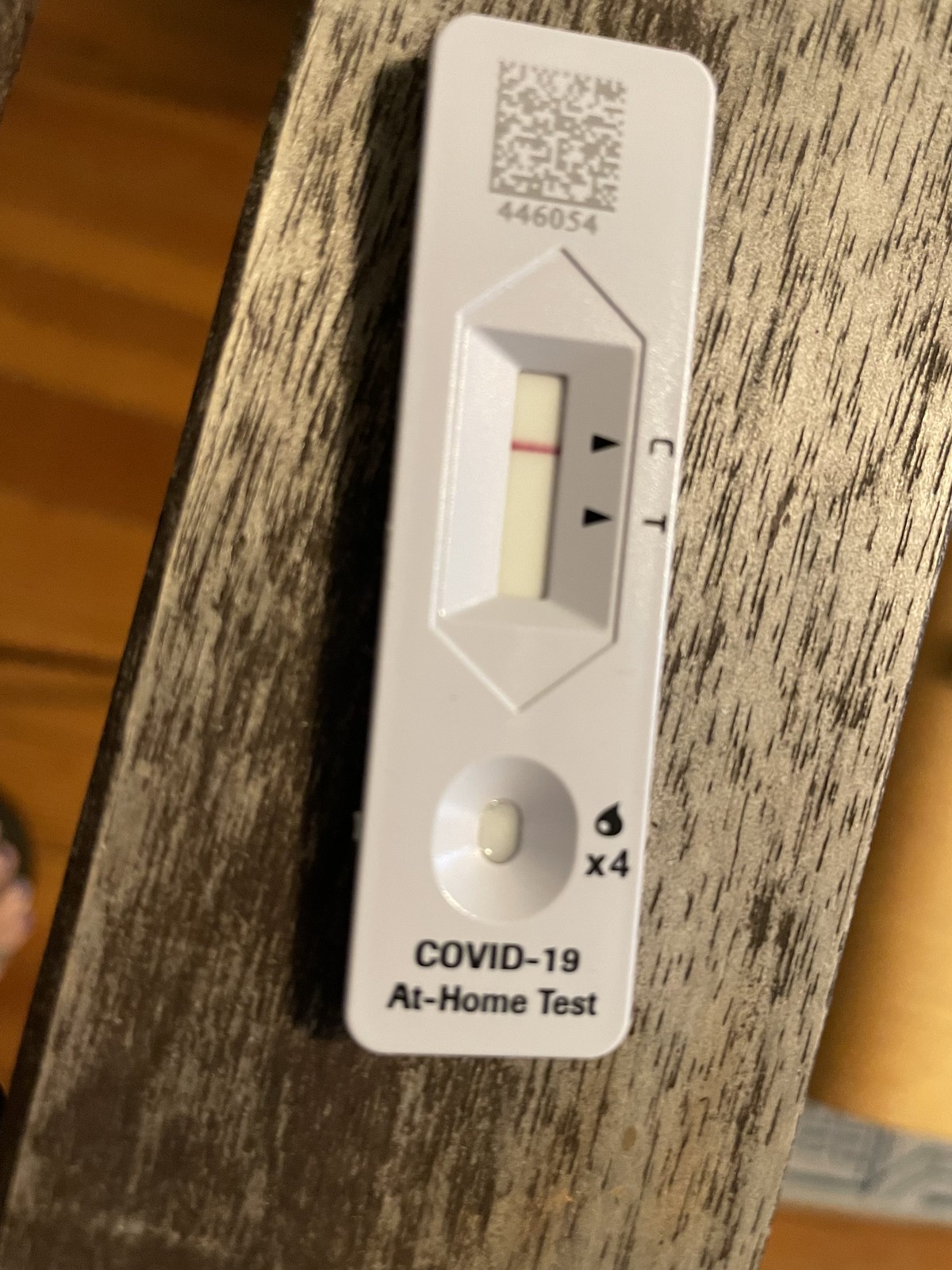The photograph showcases a COVID-19 at-home test encased in white plastic. At the top of the test cassette is a prominent QR code. Below the QR code is a small, vertical rectangular window displaying a single horizontal red line next to a black triangle marked with the letter "C." This indicates the control line. Beneath it, another black triangle marked with the letter "T" signifies where the test result line would appear, though no red line is present, indicating a negative result for COVID-19.

Further down the cassette, there is a small, round well with an oval-shaped base that appears glistening, likely due to the presence of a liquid sample. Adjacent to this well is a black icon depicting a drop, alongside the text "x4," suggesting the number of drops required.

The white plastic cassette is set against a wooden board, which appears to be elevated. In the background, parts of a tiled floor are visible, along with the toes of an individual wearing a black slipper, adding a touch of human presence to the scene.